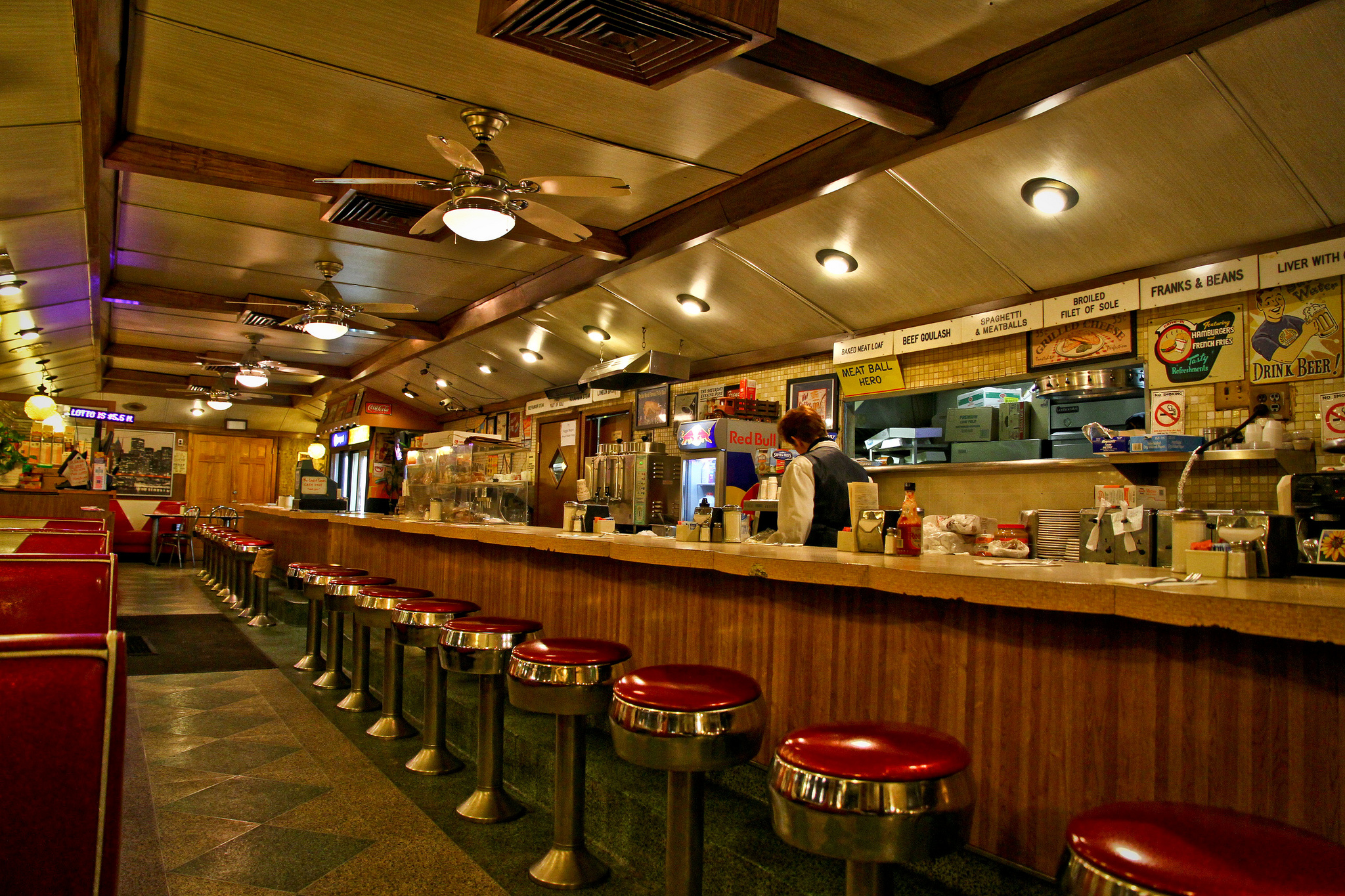The photograph captures the interior of a retro diner, exuding a classic charm with its shiny, red, attach-to-the-floor barstools and red-and-white booths on the left side. The long, brown counter, adorned with ketchup and other condiments, features paneling on its side and is fronted by barstools that have a chrome rim and a dark gray stand. The environment is brightly lit by multiple circular lights and cooled by the four ceiling fans on the ceiling. Behind the counter stands a waiter with short brown hair, dressed in a white long-sleeve shirt and a black vest, looking at the menu. In the background, the menu boards display a variety of hearty diner favorites, including spaghetti and meatballs, beef goulash, broiled fillet of sole, franks and beans, livert with onions, meatball hero, and baked meatloaf. A Red Bull refrigerator and a coffee machine are visible, along with a window to the kitchen and two double doors leading to the back. The floor is a mix of brown and gray tiles, adding to the diner’s nostalgic feel. Despite the inviting setup, the place is vacant, suggesting it might be late at night.